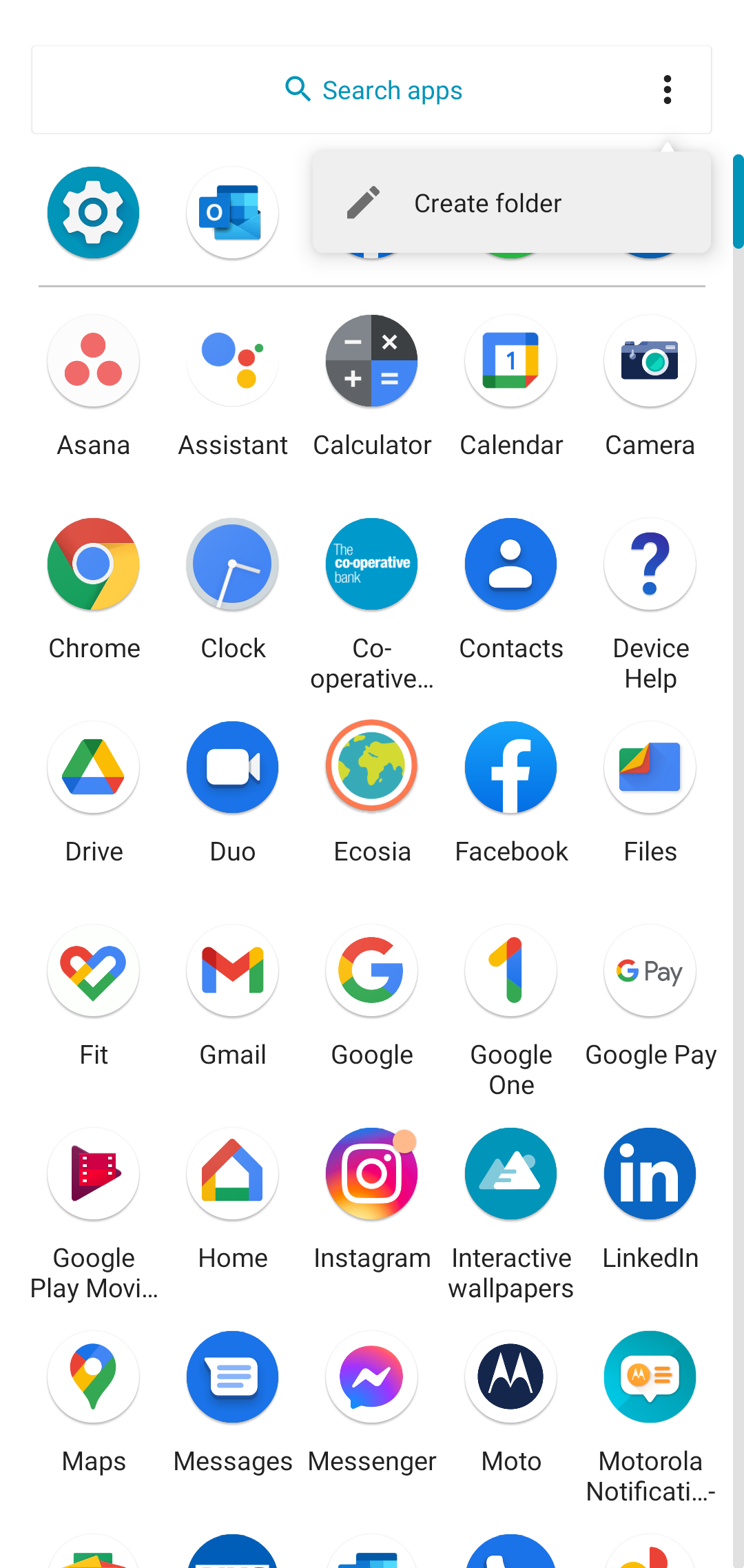In this image, we see a meticulously detailed screenshot of a smartphone’s home screen, prominently displaying its assortment of applications. At the top of the screen, a white search bar labeled "Search Apps" invites the user to quickly locate installed applications. Directly beneath this search bar is a pop-up box with the text "Create Folder," suggesting that the user is in the process of organizing apps into a new folder.

The applications are arranged in a grid format. Starting from the top left and moving across to the right, the first row contains the icons for Asana Assistant, Calculator, Calendar, and Camera. 

The second row features Chrome, Clock, Cooperative, Contacts, and Device Help.

Descending to the third row, we see Drive, Duo, Ecosia, Facebook, and Files.

The fourth row includes Fit, Gmail, Google, Google One, and Google Pay.

Further down, the fifth row displays Google Play Movies, Google Home, Instagram, Interactive Wallpapers, and LinkedIn.

Finally, the sixth row contains Google Maps, Messages, Facebook Messenger, Moto, and Motorola Notifications, indicating that this is likely a Motorola (Moto) phone given the presence of Moto-specific applications.

The screenshot collectively provides a comprehensive overview of the diverse apps installed on the device, ranging from productivity tools and social media platforms to essential Google services and device-specific applications.